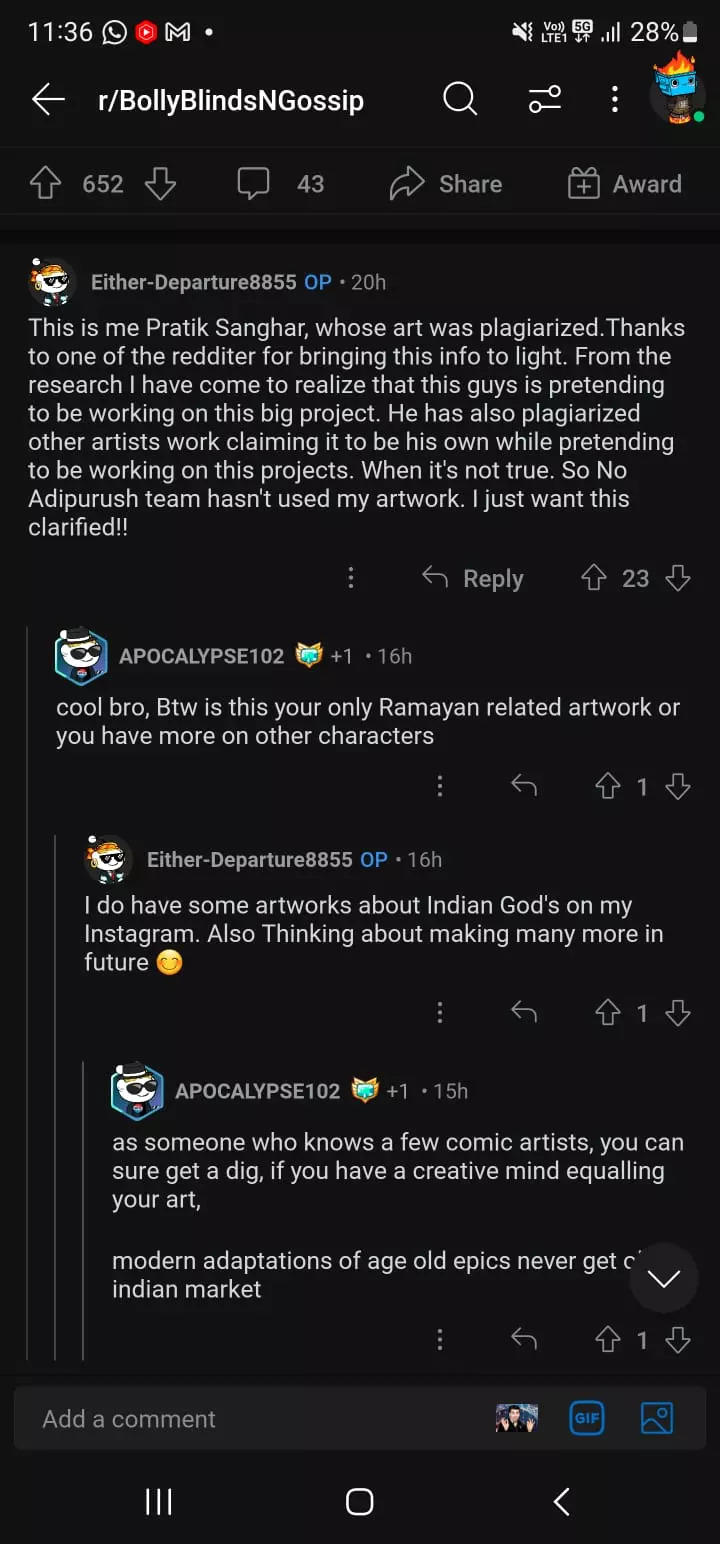In this image, there is a screenshot from a Reddit post made by the user "eitherdeparture." The post reads:

---

"This is me, Barak Chigar, whose art was plagiarized. Thanks to one of the redditors for bringing this info to light. From the research, I have come to realize that this guy is pretending to be working on this big project. He has also plagiarized other artists' work, claiming it as his own while pretending to be working on this project, which is not true. So no, 88pushteam hasn't used my artwork. I just want this clarified."

---

The poster, Barak Chigar, appears to be expressing frustration over his artwork being plagiarized and falsely credited to someone else. The post also clarifies that the group "88pushteam" has not used his artwork.

Below the main post, there are a few responses from other Reddit users. One response reads:

---

"Cool, bro. By the way, is this your only Ramanan-related artwork, or do you have more other characters?"

---

Barak Chigar replies:

---

"I do have some artworks about Indian gods on my Instagram, also thinking about making many more in the future."

---

Another reply says:

---

"As someone who knows a few comic artists, you can sure get a gig. If you have a creative mind equalling your art, modern adaptations of old-age epics never get old in the Indian market."

---

The screenshot highlights the post and comments in Reddit's dark mode, displaying white text on a black background. This provides a clear view of the ongoing conversation about art plagiarism and Barak's future artistic endeavors.